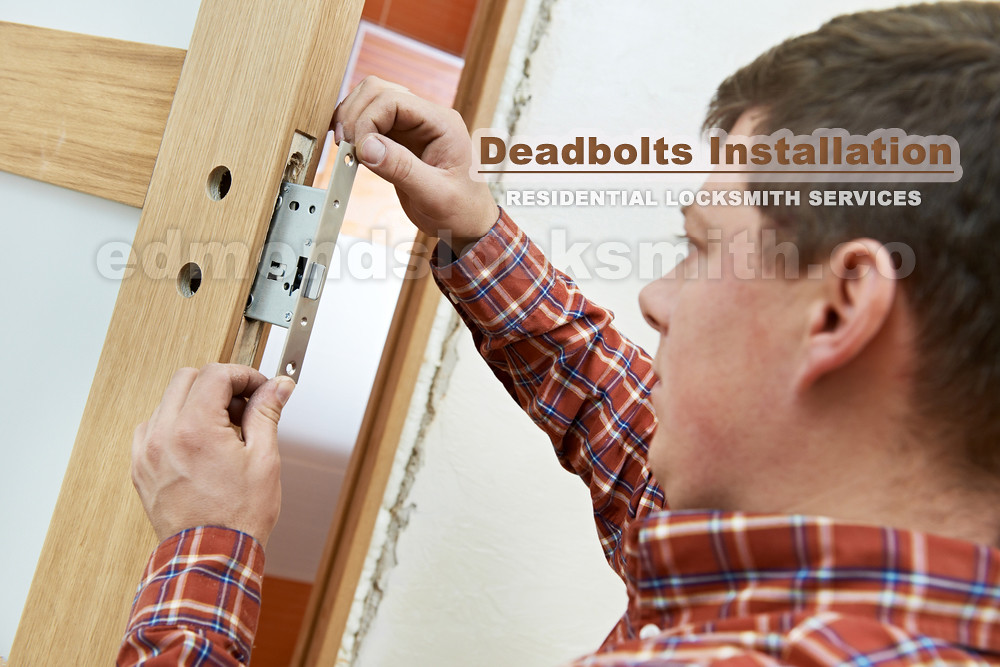In this detailed image, a man with short brown hair and light Caucasian skin is seen installing a silver steel deadbolt into a wooden door with white panels. He is wearing a distinct burnt orange or red plaid shirt with blue and yellow lines. The man is positioned to the right side of the photo, concentrating on pushing the deadbolt into the doorframe. The door itself is light-colored wood with white panels at the top and bottom, and a single wooden piece across the middle. A plain white wall serves as the backdrop. Overlaid on the photo, in translucent lettering, is the watermark "EdmondsLocksmith.co," and above the man's head, in orange and white text, are the words "Deadbolts Installation" and "Residential Locksmith Services," indicating the nature of his work.